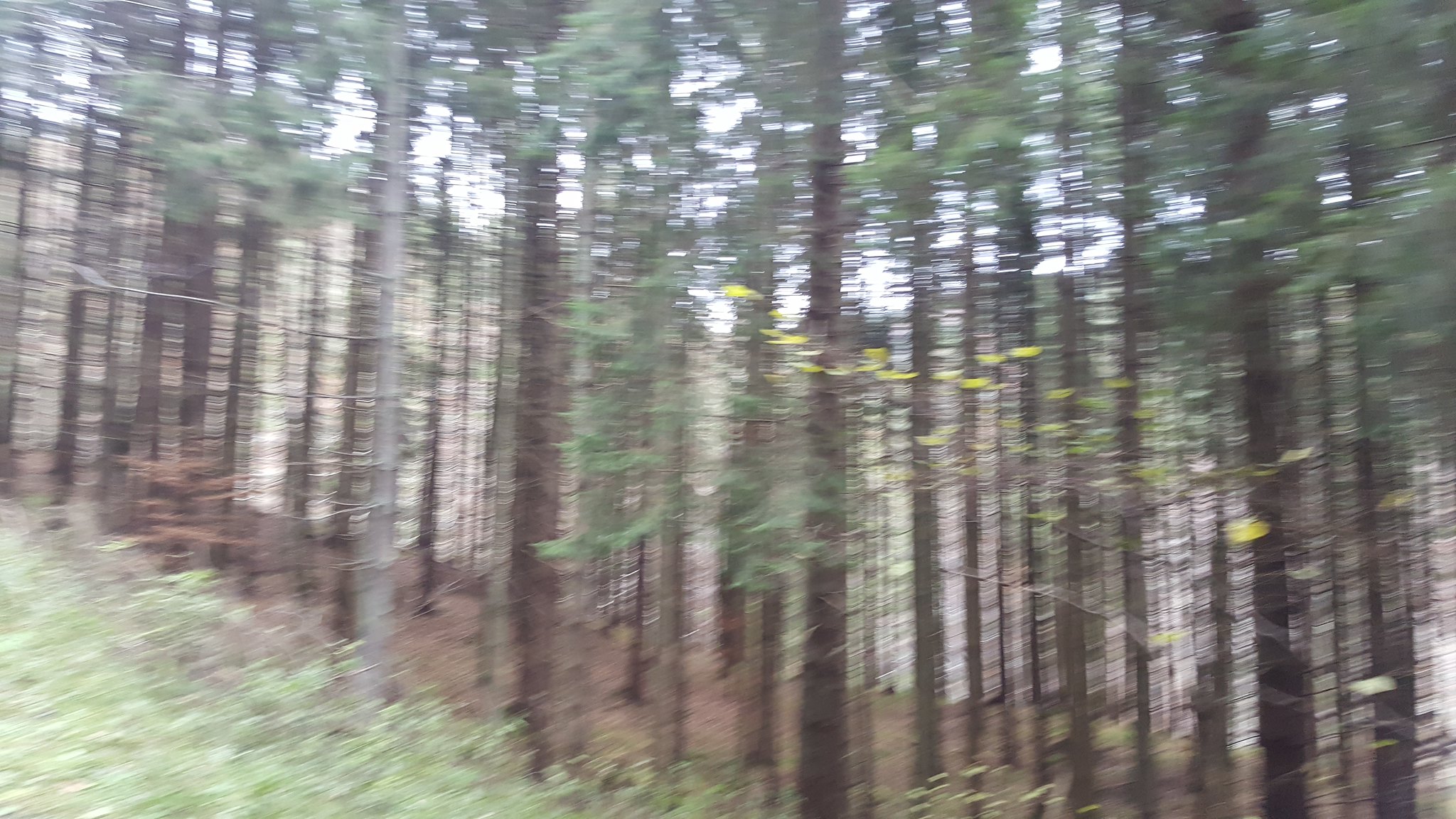A blurry photograph captures a dense woodland scene. Slender, tall trees dominate the frame, standing closely packed together and adorned with green leaves. The image lacks sharpness, making finer details difficult to discern. Amongst the trees, hints of vibrant yellow blooms can be spotted, suggesting the presence of tall wildflowers interspersed within the grove. The forest floor appears a contrasting brown, likely covered with a layer of fallen leaves or underbrush. Beyond the boundary of trees lies an expanse of greenery, possibly tall grass or a mix of wildflowers, adding texture to the landscape. Above this verdant scene, a daytime sky with patches of blue is visible, accented by a scattering of white clouds.